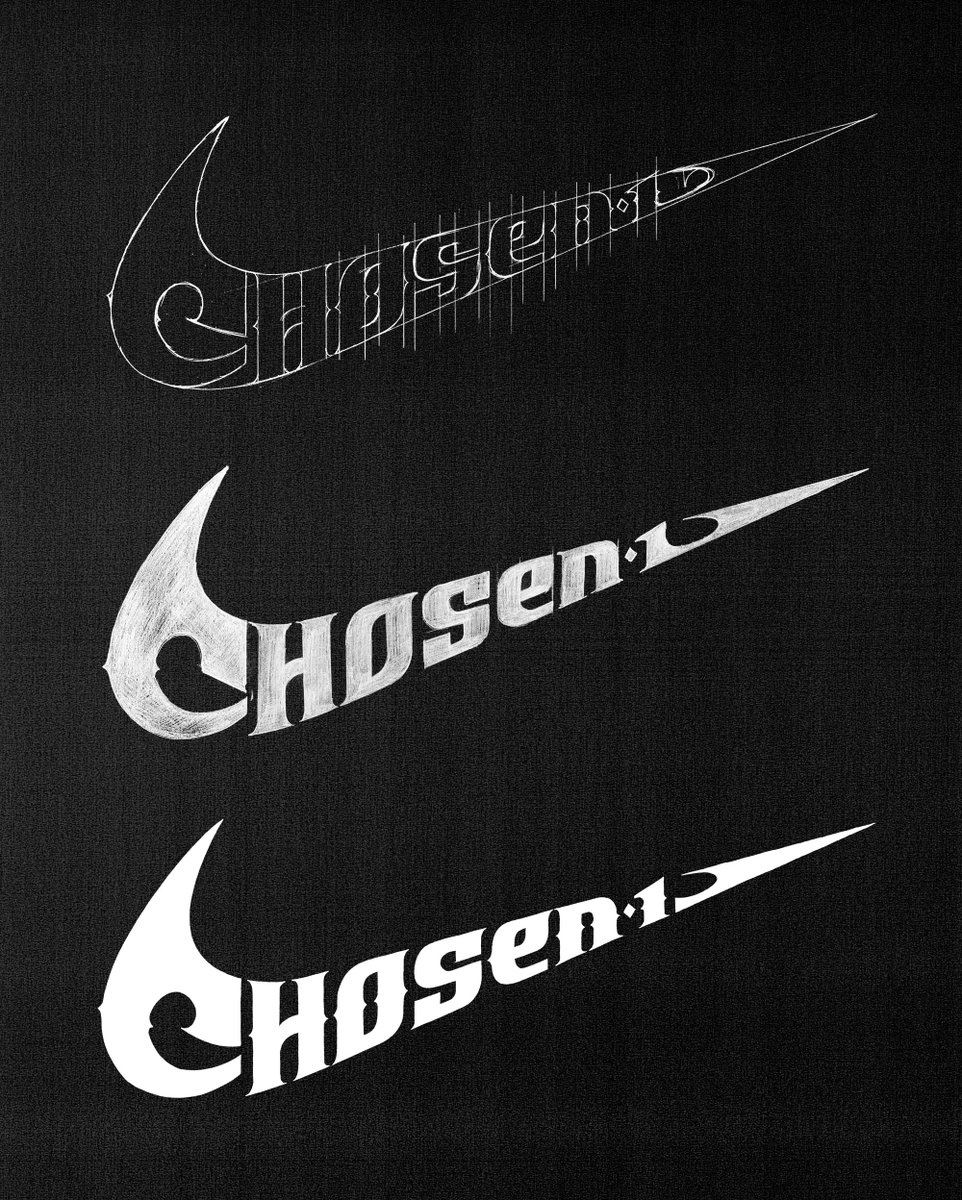This vertical digital image features a conceptual rendition of the Nike Swoosh logo against a black background. The design showcases three iterations of the Swoosh, arranged from top to bottom, demonstrating a creative process. The word "CHOSEN 1" is prominently incorporated within each Swoosh.

At the top, a minimalist Nike Swoosh is defined by a thin white outline, with the letters "C-H-O" horizontally aligned and "S-E-N" slanting upwards. The word "CHOSEN 1" is intricately placed inside the Swoosh, enclosed by white lines extending to a point beyond the text.

The middle iteration features a partially completed Swoosh, filled with solid white but accented by black smudges, resembling chalk on a blackboard. Here, "CHOSEN 1" appears unfinished, adding an evolving visual depth.

The final Swoosh at the bottom is filled with a bright, solid white, showcasing "CHOSEN 1" in its finished form. Notably, small shapes cut into the Swoosh add subtle complexity, emphasizing the detailed artistry of the piece.